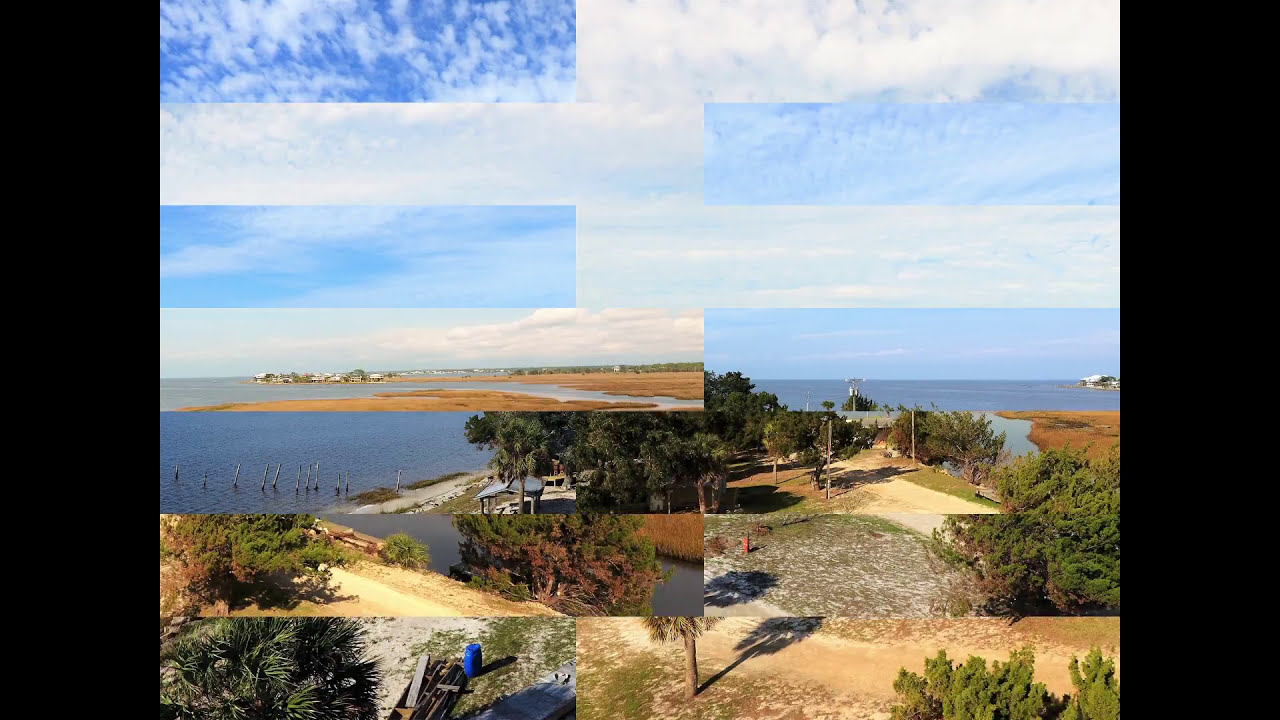The image depicts a sophisticated collage, meticulously crafted by alternating segments of two photographs. The overall composition is a horizontal rectangle, with the top portion dominated by a cloudy sky, tinged with light blue and gray hues. The left-hand side primarily showcases an ocean scene with a grayish sky and sparse clouds, transitioning into a coastline that features patches of land in the distance. Interspersed within this scene are fragments of a muddy, reddish-brown road flanked by trees, creating a complex, alternating pattern with the ocean segments.

In the central area, there's a highlighted square spot that further emphasizes the abstract nature of the collage. The horizon line is punctuated by a body of water and trees, adding depth to the composition. On the right-hand side, the lower sections reveal more of the road leading towards the ocean, accentuated with trees and additional land elements. There is also mention of a pathway to a house and components like buoys in the lake and a green or blue trash can.

The setting is clearly outdoors, captured during daytime, and blends elements of serene natural landscapes—a lake, an ocean, trees, and a road—into an intricate, visually-stimulating mosaic. The colors range broadly from blue, light blue, gray, white, to dark green, orange, and reddish-brown, creating a vibrant yet harmonious palette.